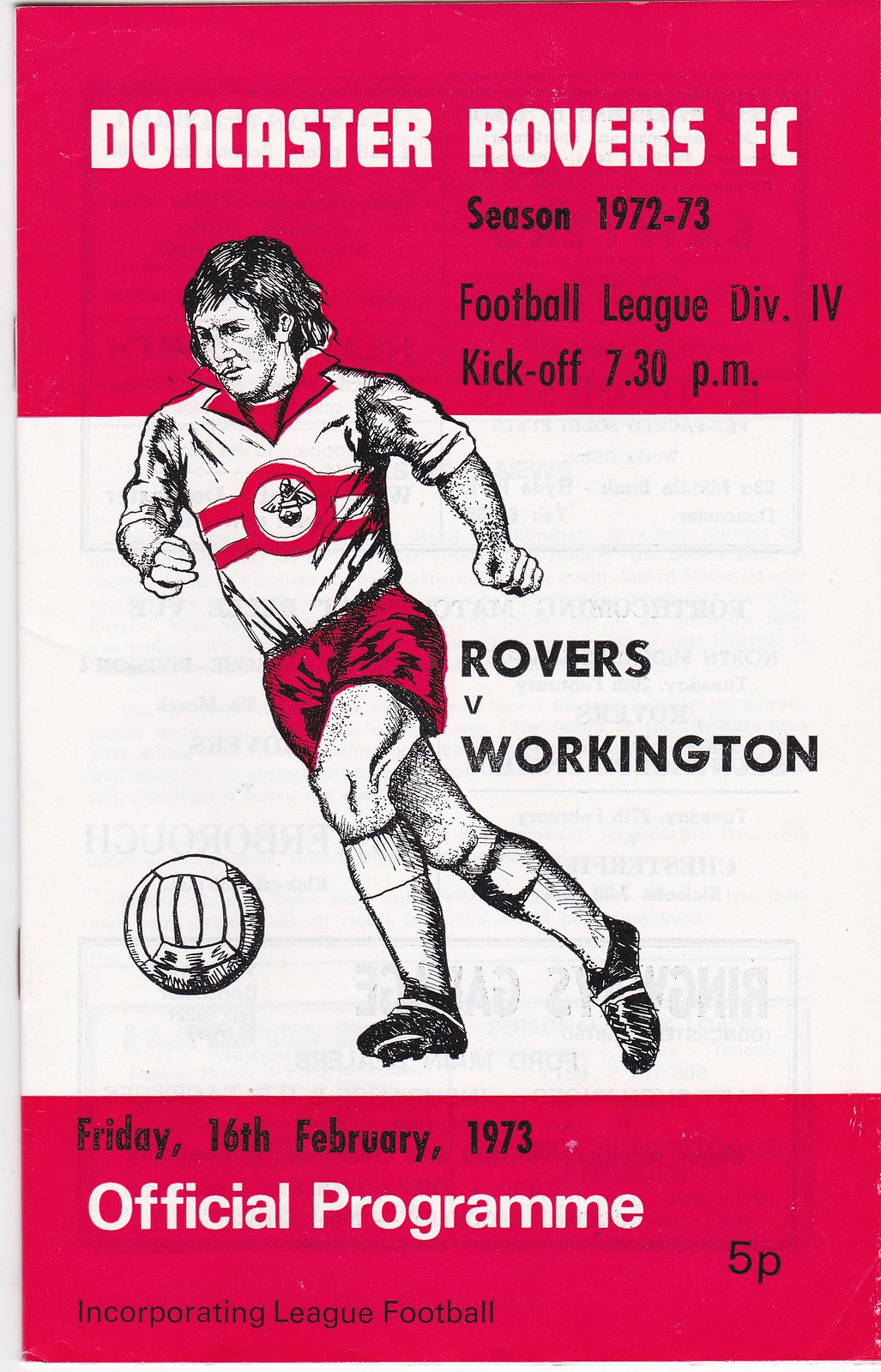This image is the cover of an official program for a football (soccer) game, showcasing a red, white, and black design. At the top, in bold white text on a red background, it reads "Doncaster Rovers FC." Below this, in black text, it details the match specifics: "Season 1972-73, Football League Division 4, Kickoff 7.30pm, Rovers vs. Workington." The centerpiece of the cover features an illustration of a soccer player with white skin and dark hair, wearing the Doncaster Rovers jersey—white with red stripes and a circular team logo, a red collar, red shorts, white socks, and black shoes—kicking a soccer ball about knee height. The bottom red section of the cover states, "Friday 16th February 1973, Official Program, Incorporating League Football," priced at 5 pence.